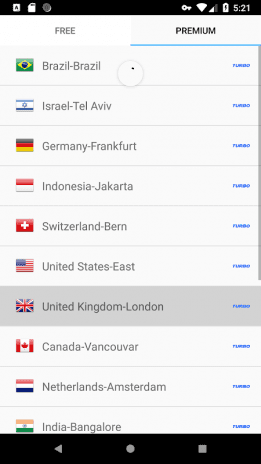A cell phone screen displays a website with the current time shown as 5:21 PM and the battery icon nearly full, indicated in white. The status bar shows a strong connection signal. At the top of the screen, there are two options: "Free" on the left and "Premium," which is underlined, on the right. Beneath these options is a blue navigation bar. 

The main content below the navigation bar lists various global locations. The countries and cities listed include:

- Brazil
- Israel (Tel Aviv)
- Germany (Frankfurt)
- Indonesia (Jakarta)
- Switzerland (Bern)
- United States (East)
- United Kingdom (London)
- Canada (Vancouver)
- Netherlands (Amsterdam)
- India (Bangalore)

Next to each location, there is a blue icon that likely indicates "Premium," consistent with the underlined "Premium" option above. The list gets cut off beneath "India (Bangalore)," suggesting that there is more content to scroll through. On the right side of the screen, a vertical gray scrollbar allows for further navigation of the page's content.